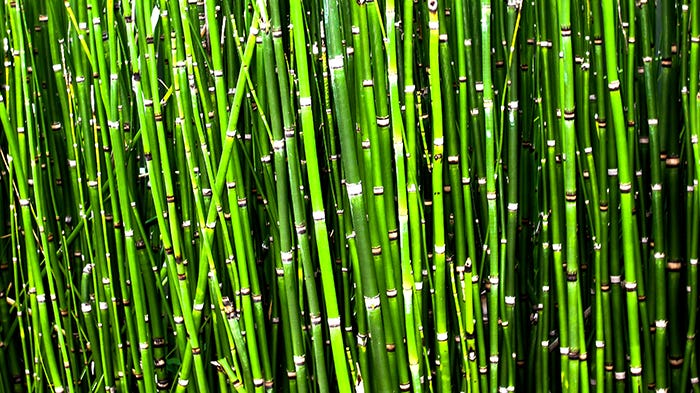This image captures a verdant field of bamboo, with densely packed stalks stretching vertically from the bottom to the top of the frame. The bamboo appears in varying shades of green, ranging from a luminous lime green in the foreground to darker hues further back. Each stalk is segmented with white or black lines approximately every inch or so, which give an impression of glowing light. These rings, evenly spaced, mark the growth joints of the bamboo. While most of the bamboo shoots stand upright, a few pieces lean diagonally to the right, adding a dynamic element to the composition. The overall effect is a rich tapestry of green bamboo, evoking both the natural order and slight disorder within the dense thicket.